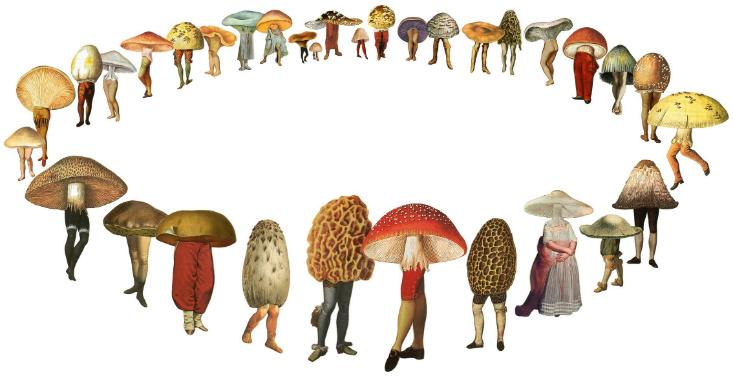This lively, cartoonish graphic presents an imaginative scene featuring approximately 30 anthropomorphic mushrooms and toadstools standing in a circle against a blank white background. Each mushroom boasts a distinct appearance, with caps of various shapes and colors—ranging from a classic red cap with white spots to dried, white, and orange varieties. The mushrooms are characterized by their human legs, adorned in a variety of attire such as black shoes, socks, colognes, and diverse clothing items like red shirts, brown shorts, and even some with bare legs. One mushroom on the right appears to be dancing, while others, hampered by their broad caps, make do with limited space. Smaller, child-like mushrooms add to the whimsy of the scene, enhancing the overall playful and adorable atmosphere.